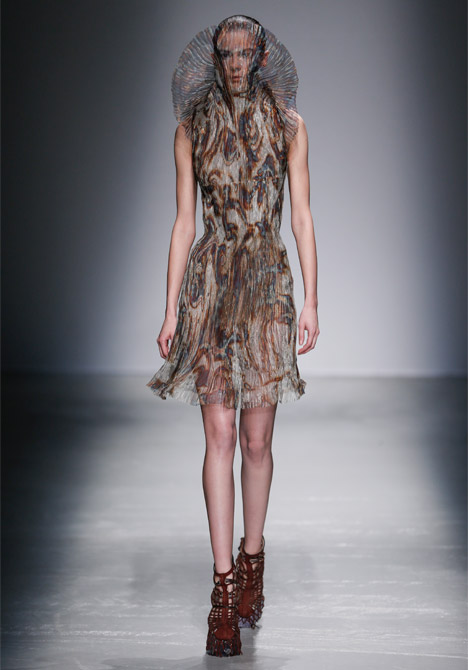A tall, extremely thin, Caucasian model with a shaved head is walking down a gray runway, framed by shadowy gray walls and vignetted lighting that highlights her striking appearance. She wears an avant-garde ensemble featuring a sleeveless, partially see-through dress that ends just above her knees. The dress, made of a wispy, reedy material reminiscent of a transparent gauze or potato cloth, features an intricate pattern of white and rusty dark brown swirls and splotches. Covering her face and extending down to her shoulders is a tightly fitted, see-through veil, complemented by a fan-like structure made of the same material that extends behind her head in a half-circle. Completing the look, she steps confidently in high-heeled boots with black mesh and red leather straps.